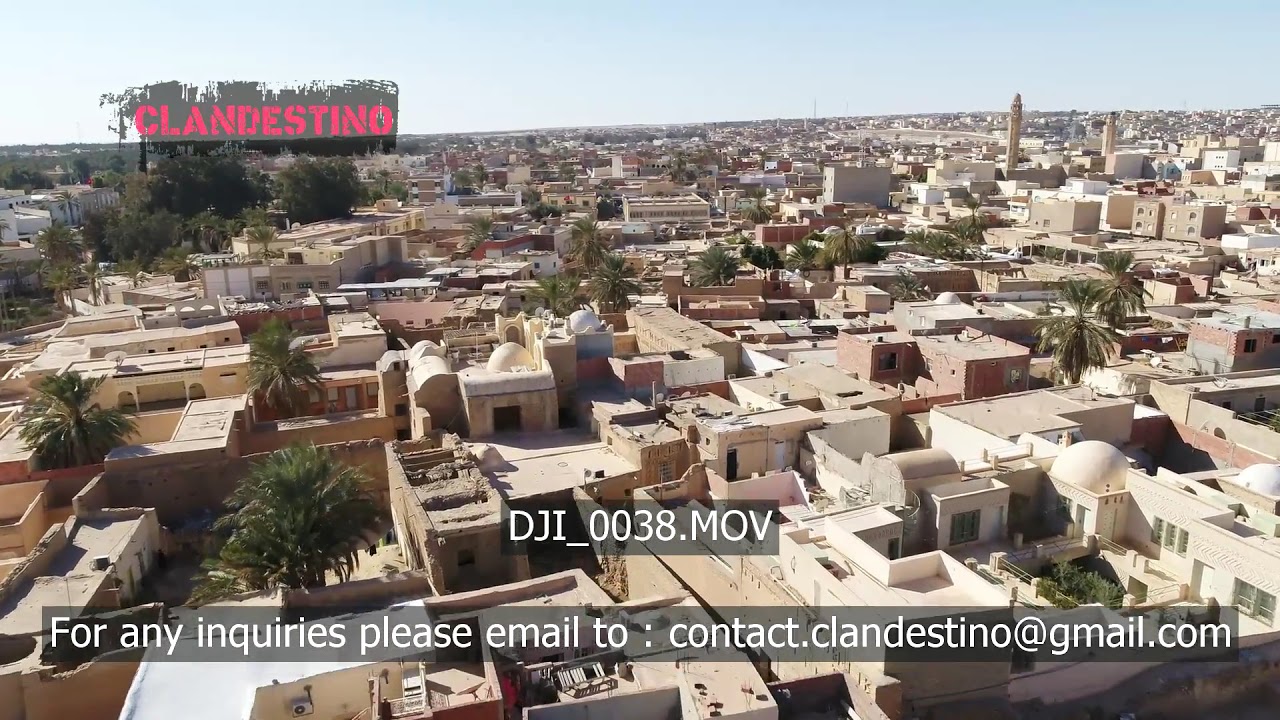This vibrant, full-color photograph captures an expansive aerial view of a densely built town, presumably located in the Middle East. Bathed in bright sunlight under a clear, light blue sky, the town features closely packed buildings, all constructed in a uniform light brown or tan color. Distinctive architectural elements include numerous domed roofs adorning many of these structures, which generally appear to be low to the ground. Some buildings exhibit minimal openings, with some even lacking windows. The courtyards of these buildings are punctuated with palm trees that add a touch of green to the earthy tones. At the upper left corner of the image, a gray rectangular area is overlaid with red text reading "CLANDESTINO." Towards the bottom center, digital text reads, "DJI_0038.MOV," followed by an inquiry email, "contact.clandestino@gmail.com." The entirety of the arrangement suggests that the photo may be part of an advertisement for "CLANDESTINO."